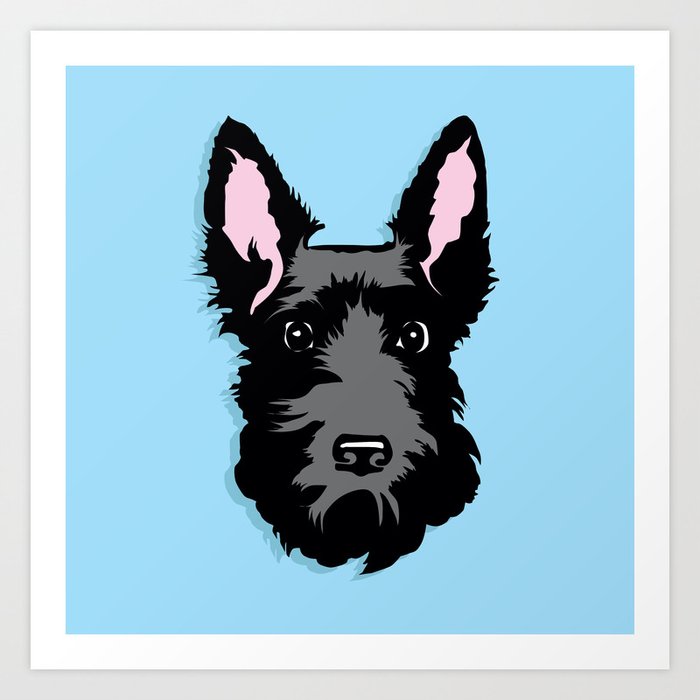The image is a digitally-produced, square portrait of a Scottish Terrier's head set against a light blue background. It features a meticulously detailed depiction using a color palette including black, white, gray, light pink, and light blue. The dog's black face is accented with gray, and it has striking light pink inner ears. The eyes are wide open and black, showing a stark contrast against the background. The nose, also black, is prominently positioned at the center of the face. The head is framed by subtle detailing of darker blue around its edges, enhancing its dimensionality. The overall image is enclosed within a light gray square outline, which is then further bordered by a white square. There is no text or additional imagery, making the focus solely on the dog's face. The artistry leans towards a clean, bright, and clear digital style, suggesting that it could have been created by either an amateur or someone with an artistic background.